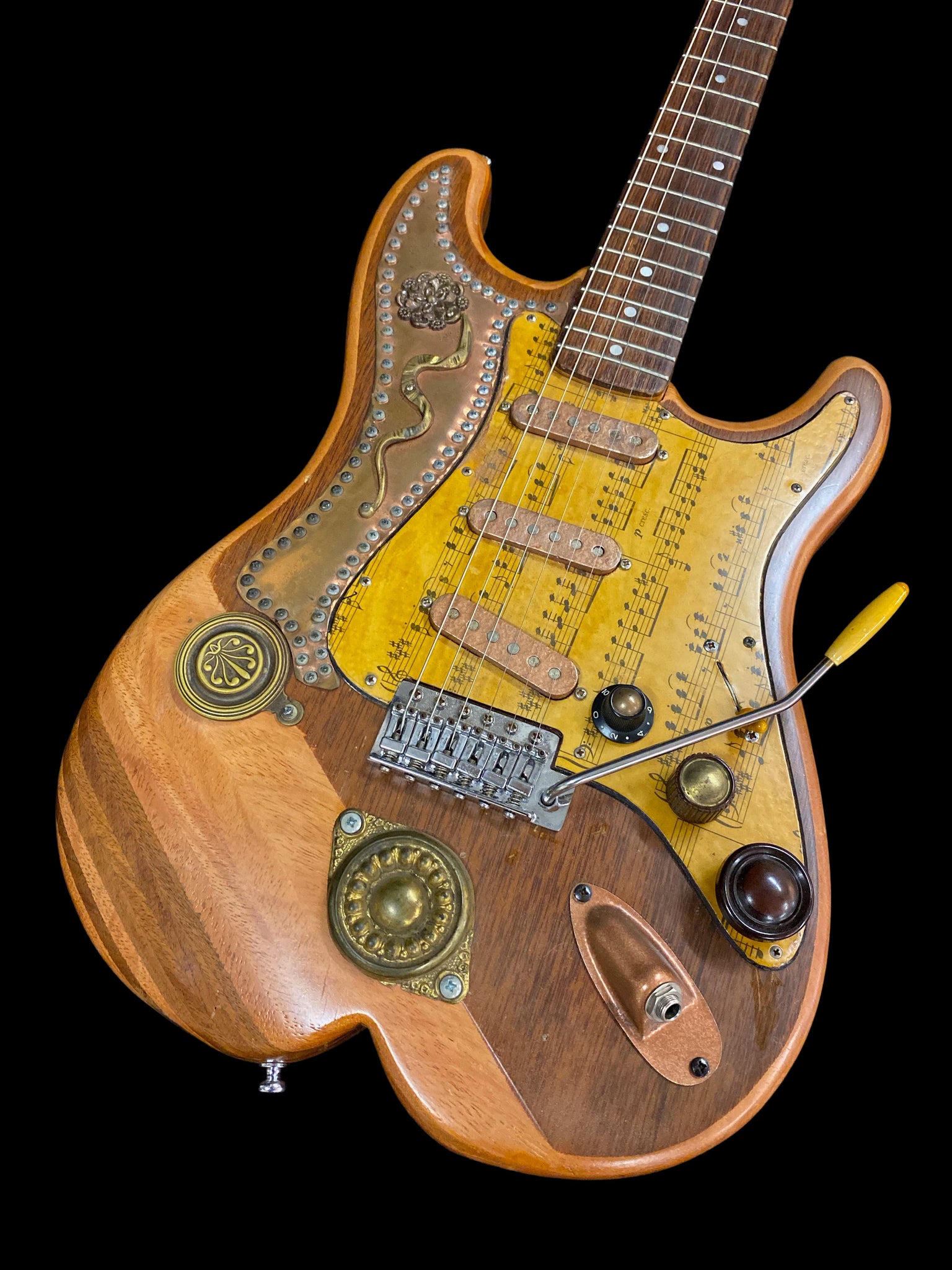This is a studio photograph showcasing a uniquely designed electric guitar against a pitch-black background. The guitar's body, crafted from a variety of shiny wood types, features a striking combination of colors and materials. The base is a lighter brown, adorned with a central inset of darker wood. Embedded within this central section is a yellowish wood panel, intricately inscribed with musical notation in black. Decorative brass elements, including a prominent 3D snake emblem and wavy brass plates with silver rivets, enhance the guitar's ornate appearance. The guitar strings are metal, and the tremolo bar is tipped with a yellow piece. The neck of the guitar, which extends out of the frame to the top right, is dark brown and features the continuation of the guitar's intricate design. The right side of the body also includes several bronze or brown knobs and an electrical input for an amplifier.